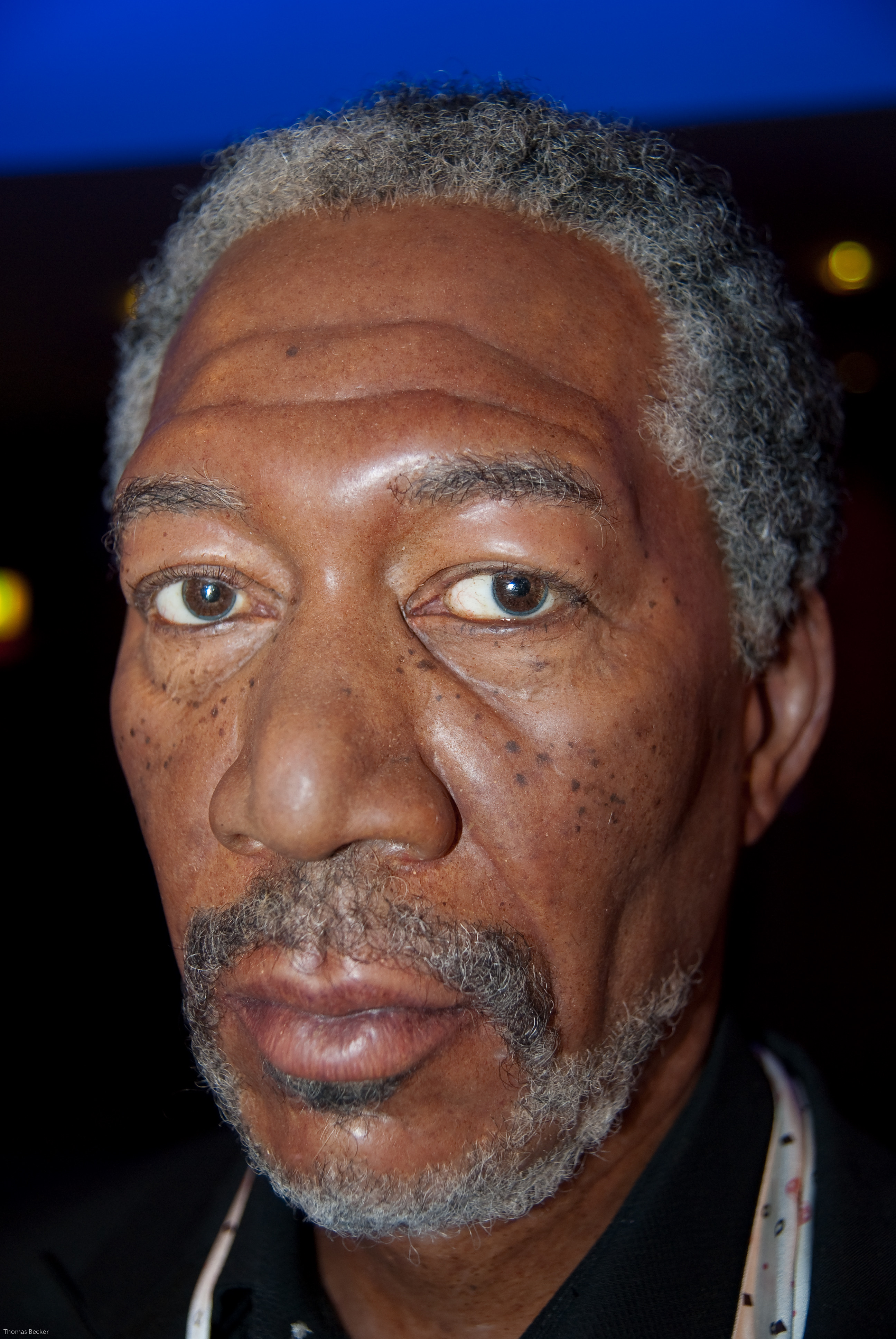The photo captures a high-definition close-up of the esteemed actor Morgan Freeman, a black male likely in his early 70s. His hair, a mix of gray and white, is cut fairly short, complementing his neatly trimmed mustache and beard. Freeman's brown eyes stand out amidst the subtle constellation of freckles that dot the area around them. Illuminated by a strategic light source, his facial features are prominently highlighted against a dimly lit background. He is adorned in a white, thin scarf paired with a dark blue or black collared T-shirt. The defined structure of his face, including noticeable cheekbones, suggests he is slightly clenching his jaw, with his lips firmly closed, presenting a contemplative expression.